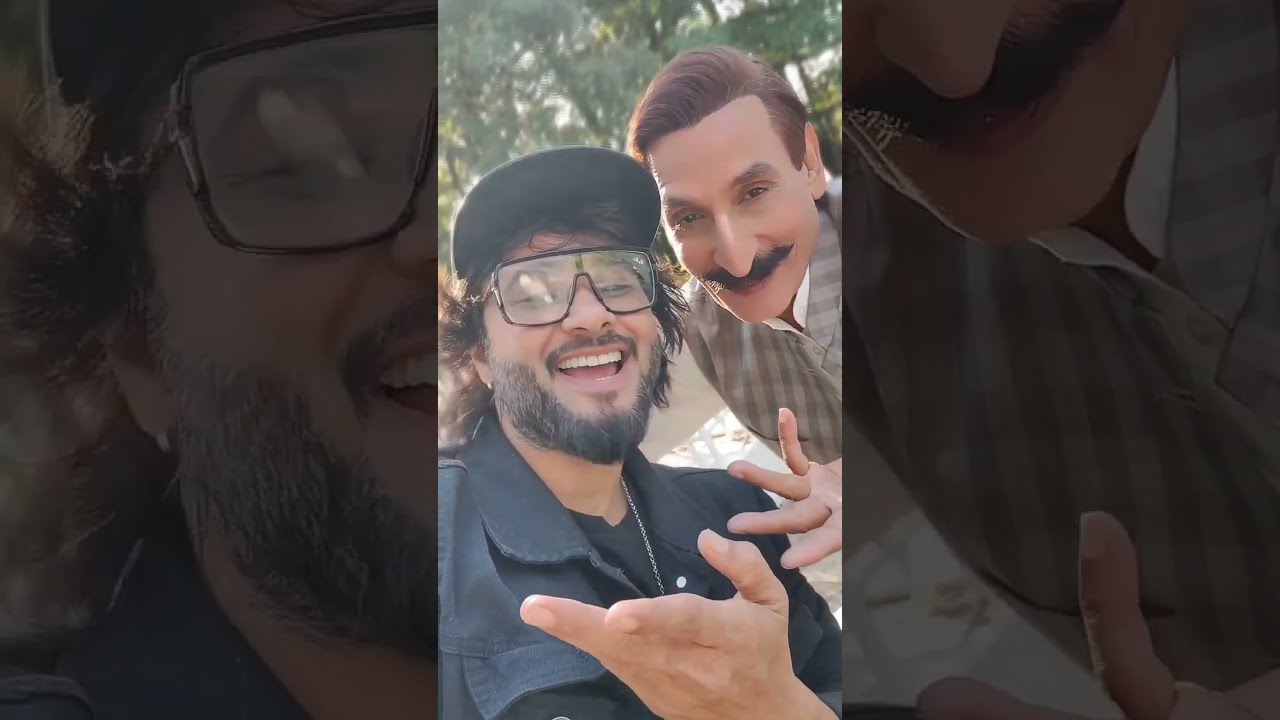The photograph features two men posing together in the center. The man on the left, with tan skin and a smiling expression, wears a black baseball hat with the bill just visible. His dark, shaggy hair peeks from beneath the hat, and he sports large, square-shaped black frames with clear lenses. His facial hair consists of a mustache and a short beard. He's dressed in a black collared shirt layered over a black t-shirt, with a hand posed palm up towards the camera. Next to him on the right is a man with combed-over light brown hair. His distinctive features include a pointy nose and thick, black mustache. He wears a tan and white checkered shirt and mirrors his friend's hand gesture, also with his palm facing up. Both are smiling directly at the camera. The background is a faded, close-up version of the main image, creating a border effect on either side, and adding a layered depth to the photograph.